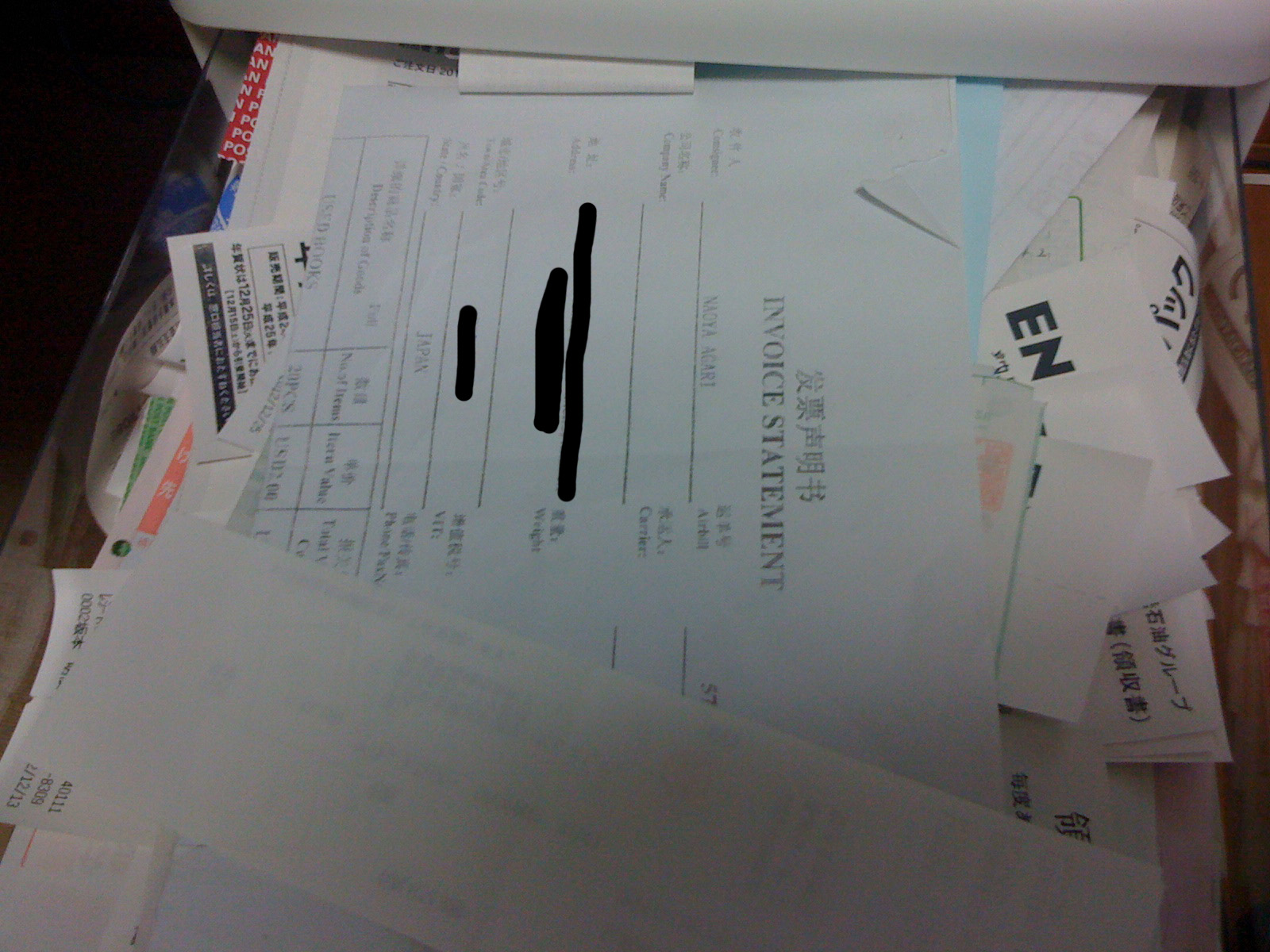The image depicts a slightly cluttered scene atop a glass-like surface, possibly a desk or drawer, filled with an array of papers varying in color, size, and type. Prominently visible is a white sheet of paper featuring Chinese writing, with the English words "invoice statement" clearly printed below. This paper includes multiple lines of notation, some of which have been redacted with black marker. Also notable are various other colored papers—red, blue, green—peeking out from underneath the main stack. In the upper left corner of the image, a dark-colored chair is partially visible, suggesting that this surface is likely part of a busy workspace where substantial paperwork is processed and stored. The overall scene gives an impression of a densely packed yet semi-organized collection of important documents, highlighting a glimpse into a meticulous and busy office environment.